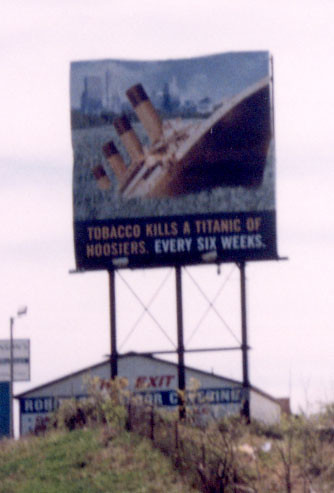A blurry, out-of-focus photograph captures a high-mounted billboard on a bright, daylight backdrop. The billboard, elevated two stories above a nearby building, prominently displays a city skyline graphic with a sinking ship. Below this imagery, a black box with bold yellow font urgently declares: "TOBACCO KILLS A TANNIC OF HOOSIERS EVERY SIX WEEKS," with "every six weeks" emphasized in white. The building behind the billboard has a partially obscured sign reading "EXIT" in red font, hidden among the trees. The sky appears hazy in a white-gray hue, adding to the low-quality nature of the image.